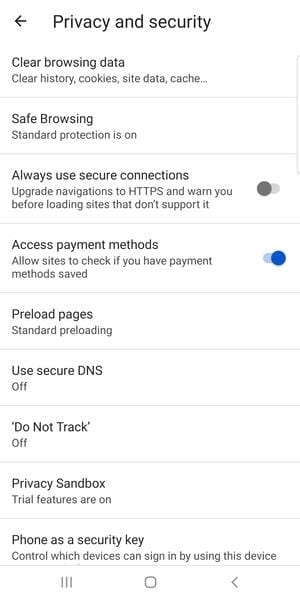The image depicts a comprehensive privacy and security settings pop-up, likely from a device's settings menu. The layout features a clean design primarily in black and white, with the exception of interactive elements like selected buttons, which turn blue when activated and remain gray when deactivated.

The options listed include:

1. **Clear Browsing Data**: Encompassing the clearing of history, cookies, site data, and cache.
2. **Safe Browsing**: Indicating that standard protection is enabled.
3. **Always Use Secure Connections**: This is unselected, meaning the feature to upgrade navigations to HTTPS and warn before loading sites that don't support it is inactive.
4. **Access Payment Methods**: This is selected, allowing users to manage saved payment methods.
5. **Preload Pages**: Indicates standard preloading is active.
6. **Use Secure DNS**: There's an option for using secure DNS.
7. **Do Not Track**: This feature is turned off.
8. **Privacy Sandbox**: Trial features are on.
9. **Phone As a Security Key**: This controls which device can be used for signing in.

The overall appearance is minimalist with a plain white background and no additional graphics or identifiers indicating the specific device in use.